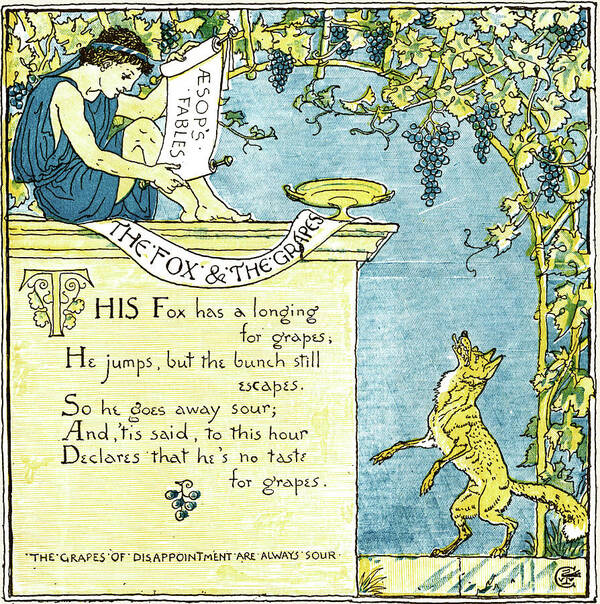This illustration is a vibrant plate from a book of Aesop's Fables, specifically "The Fox and the Grapes." The scene, resembling a fresco with Grecian elements, is dominated by a narrative inscribed on a yellow stone wall. The fable text reads: "This fox has a longing for grapes. He jumps but the bunch still escapes, so he goes away sour and 'tis said to this hour, declares that he's no taste for grapes. The grapes of disappointment are always sour."

Perched on top of this wall is a man with olive skin, dressed in a blue toga and headband, holding a scroll that reads "Aesop's Fables" in Latin. His legs extend in front of him and a yellow chalice sits near his feet. The image captures a fox, golden with white under its chin, struggling to reach bunches of blue grapes hanging from a lush grapevine that stretches over an archway. The fox stands on its hind legs on a stone path, its front legs raised, and its mouth slightly open in determination, yet the grapes remain just out of reach, symbolizing unattainable desire. On the right, a dog looks up longingly at the same scene, adding to the theme of unreachable aspirations. The entire image is detailed with green grape leaves, a stone box, and a serene blue background, creating a rich, illustrative tableau of the classic moral tale.